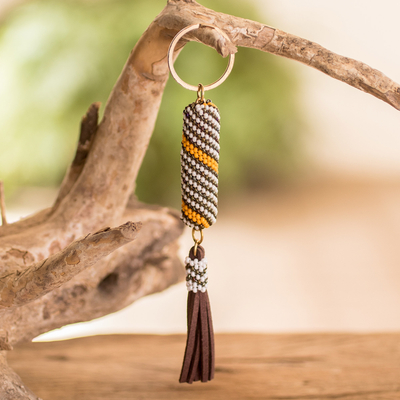The image showcases a beaded keychain hanging from a light beige, driftwood-like tree branch, carefully curated as a display holder. The keychain features a circular gold ring at the top, connected to an intricate cylindrical body adorned with a diagonal pattern of white and brown beads, interspersed with two rows of yellow beads. Below this beaded cylinder, a brown leather tassel adorned with additional beads at its attachment point hangs gracefully. The scene is set against a blurred background that hints at green foliage and concrete, positioned above a flat wooden table surface. The branch, purposefully crafted to hold the keychain, extends both vertically and horizontally, adding rustic charm to the composition.